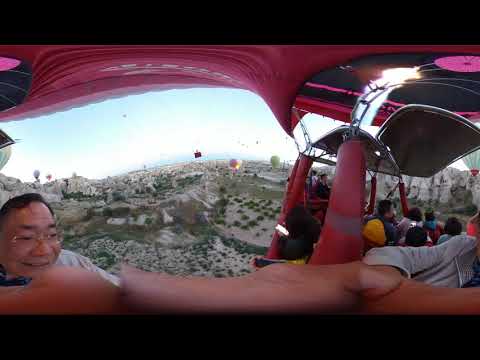In the foreground of this vibrant image, a man with short dark hair and glasses is smiling directly into the camera, situated in a red-covered enclosure that appears to be part of a ride ascending a mountainside. To his right, several people face away, absorbed in the stunning view of the landscape below. The red enclosure continues to the right, indicating multiple similar structures filled with people. 

The panoramic vista reveals a rugged terrain with brown soil dotted with green trees and shrubs, looking out over a desert-like expanse. In the distance, a series of multicolored hot air balloons float gracefully; notable ones include a pink and yellow, a green, an orange, and a white balloon. The blue sky stretches out, framing the rolling hills or mountains that recede into the horizon. Blurring the foreground, a hand reaches out horizontally across the image, adding a sense of depth and movement to the scene, which may also indicate the presence of an additional rider enjoying this popular scenic attraction.